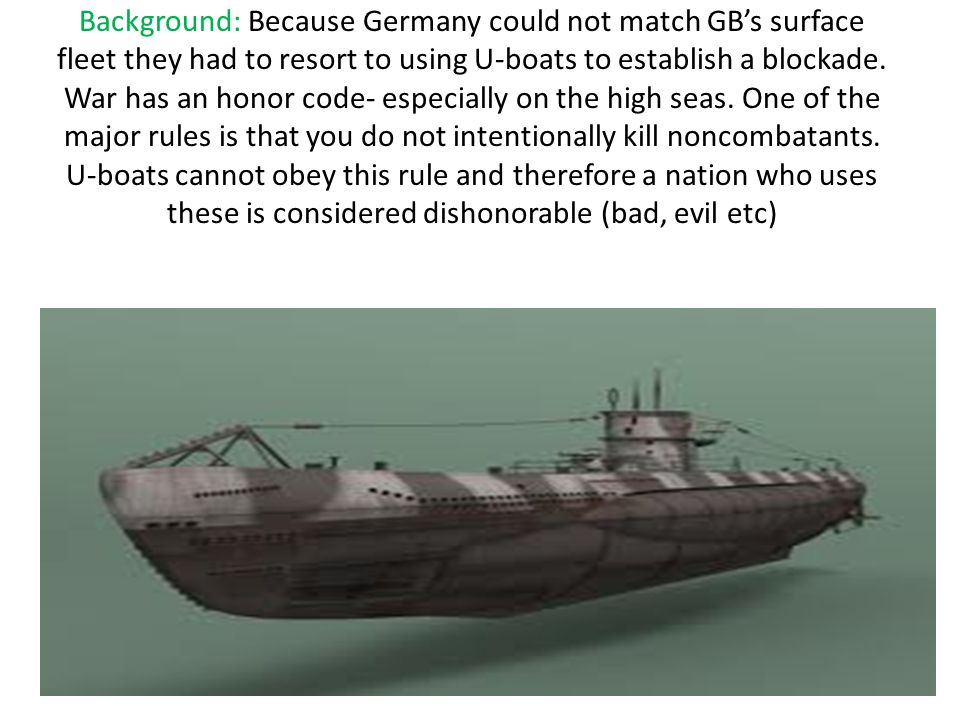This image prominently features a U-boat, depicted in varying shades of gray and dark gray, with a shadow suggesting it is illuminated from above. The U-boat appears suspended in midair against a solid gray background. Above the U-boat, a block of text provides historical context, noting that "Background," in green, explains that because Germany could not match Great Britain's surface fleet, they resorted to using U-boats to enforce a blockade. The text continues in black, explaining that war has an honor code, especially at sea, which includes not intentionally killing non-combatants. It emphasizes that U-boats, which could not adhere to this rule, rendered their use as dishonorable and, by extension, characterized the nation deploying them as bad or evil. The U-boat's appearance is described as having a dull, patchy quality with a light and dark gray color scheme.